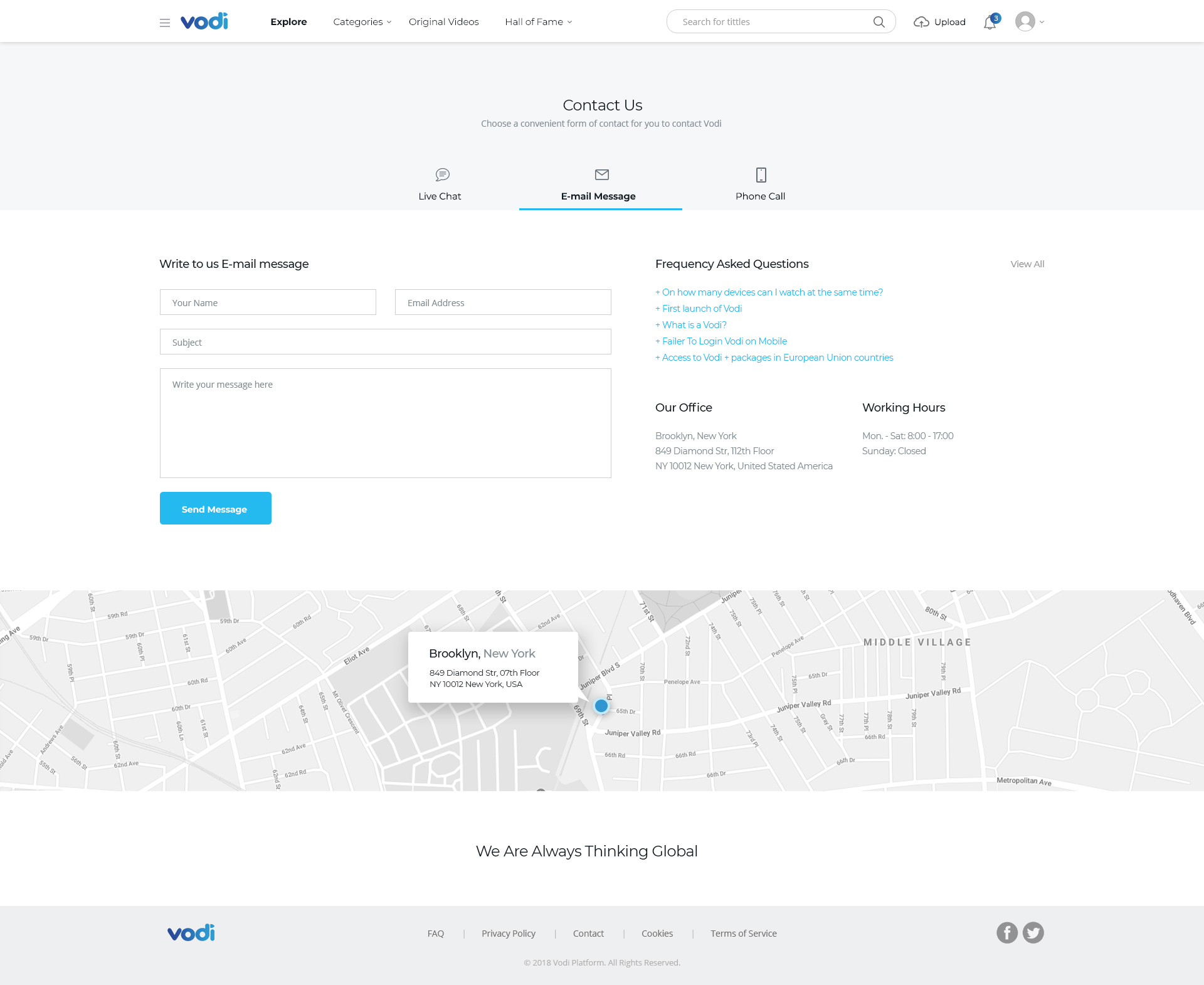In the upper left corner of the image, the word "Vodi" (spelled V-O-D-I) is displayed in a gradient that transitions from dark blue to a lighter, turquoise-blue. Beside "Vodi," there are three horizontal lines indicating a menu that can be expanded. Over to the right side of the menu, there are several navigation options: "Explore," "Categories" with a drop-down arrow, "Original Videos," "Hall of Fame" with another drop-down arrow. Further to the right is a search bar labeled "Search for Titles," accompanied by a search icon.

Next to the search bar, there's a "Cloud" icon with an arrow pointing towards it, labeled "Upload." Adjacent to this is a bell icon with a blue circle containing the number three, signifying three notifications. Finally, a user profile icon with a drop-down menu appears at the far right.

In the center of the image is a section titled "Contact Us," inviting users to choose a convenient method to contact Vodi: Live Chat, Email Message, or Phone Call. The "Email Message" option is highlighted in black bold text and underlined in blue.

On the left side, the "Write to Us" section appears, featuring a form with the following fields: "Your Name," "Email Address," "Subject," and a larger field for the message labeled "Write Your Message Here." Below this form, there's a blue button with white text that says "Send Message."

To the right of the contact form, there's a "Frequently Asked Questions" section, featuring questions with a plus sign next to each one. The questions listed include:
- "On how many devices can I watch at the same time?"
- "First Launch Vodi."
- "What is a Vodi?"
- "Failure to log in to Vodi on a mobile."
- "Access to Vodi Plus packages in European Union countries."

Below the FAQs, the company's office information is provided: 
- Location: Brooklyn, New York, 849 Diamond Street, 112th Floor, New York, 10012, New York, United States.
- Working hours: Monday through Saturday, 8:00 to 17:00, closed on Sunday.

Finally, there is a map displayed at the bottom of the image.